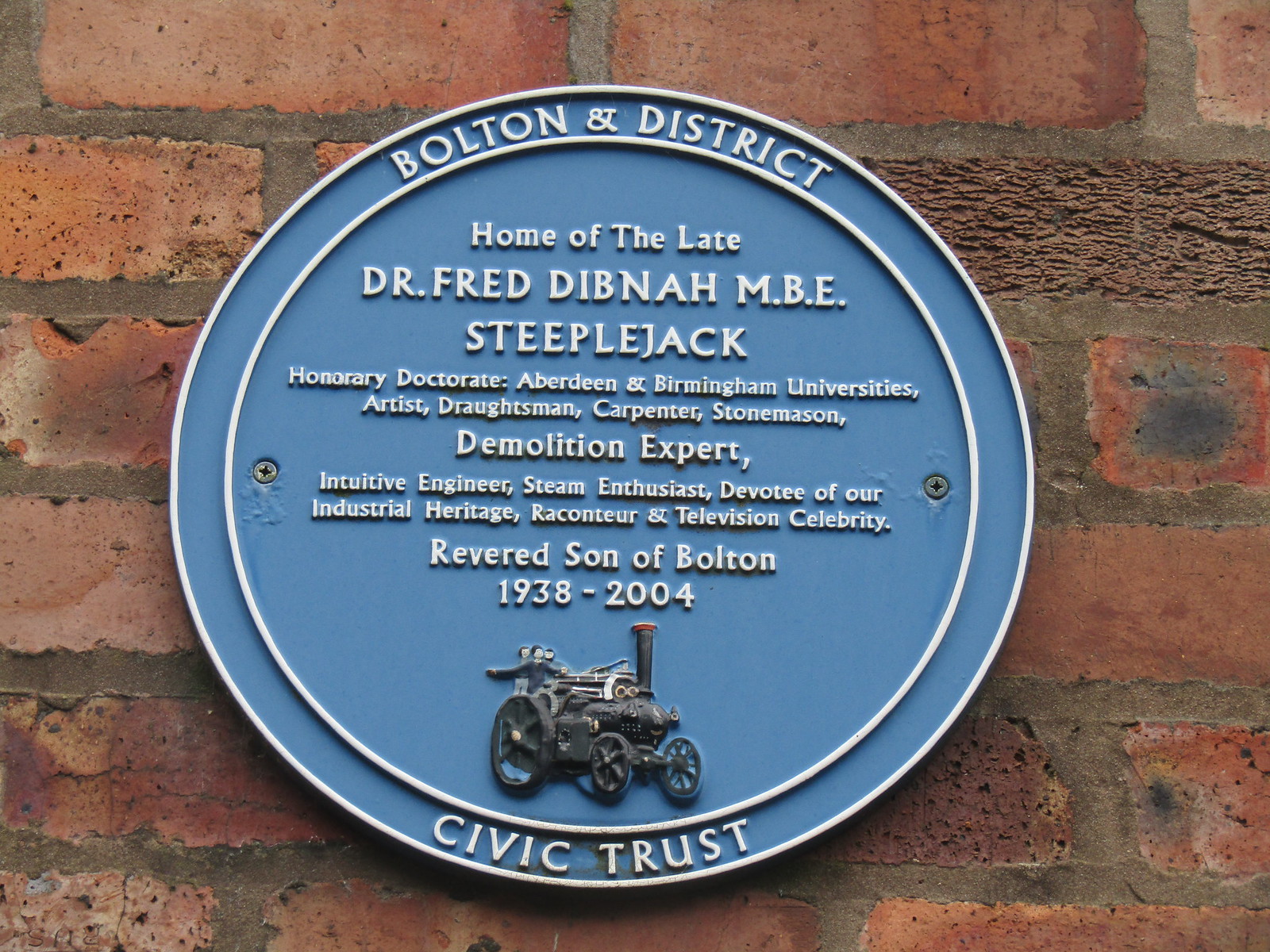The image captures a circular plaque mounted on a brick wall, commemorating the late Dr. Fred Dibnah, MBE (1938-2004), a revered son of Bolton. The plaque, presented by the Civic Trust, honors Dibnah's diverse achievements and contributions. It reads: "Bolton and District, home of the late Dr. Fred Dibnah, MBE, Steeplejack, honorary doctorate from Aberdeen and Birmingham Universities, artist, draughtsman, carpenter, stonemason, demolition expert, intuitive engineer, steam enthusiast, devotee of our industrial heritage, raconteur, and television celebrity." Below the inscription, a carved image depicts Dibnah riding an old steam-powered vehicle, accompanied by three individuals.